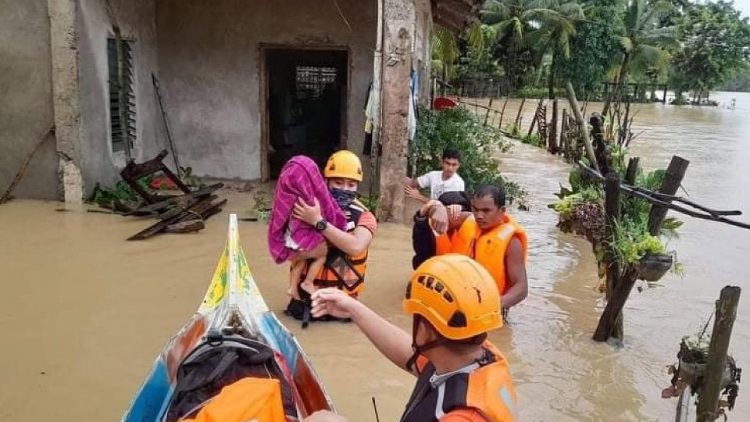In this outdoor image, a flood-ravaged tropical area is depicted. The scene is dominated by muddy, brown water engulfing both man-made and natural elements. On the right side of the image, wooden posts protrude from the murky waters, surrounded by submerged bushes and trees. 

To the left, a concrete building appears heavily damaged, with debris strewn around its entrance. The structure is constructed from mortar and stone, featuring a wooden door and a window with green blinds. Inside, the dark interior reveals rubble and wet, rotting wood.

Amidst this devastation, a rescue operation is underway. Five to six people, all wearing orange life vests and some with orange or yellow protective helmets, navigate the floodwaters. One rescuer is carrying a baby swaddled in a purple blanket, shielding her from the chaos. The rescuer has a watch on his left wrist. Nearby, a child in a white t-shirt is visible.

In the lower center foreground, the bow of a colorful canoe—painted blue, red, yellow, and brown—breaks through the water. Rescuers are packing the boat, likely to evacuate the people from the flood zone. The entire scene conveys the urgency and grim reality of a natural disaster, with the tropical environment indicating a possible location in the Dominican Republic or somewhere in Asia.